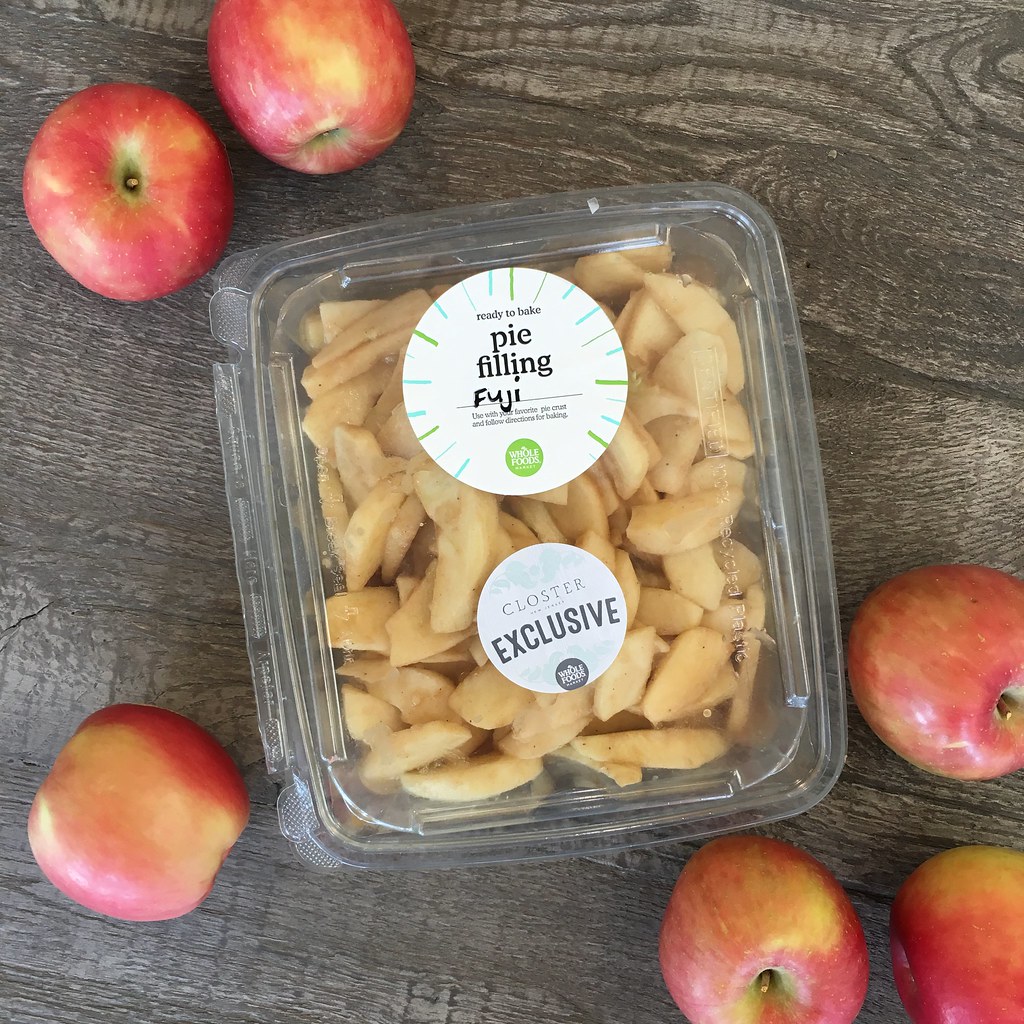A slightly tilted rectangular plastic container lies on a dark wooden surface. The container, rounded at the edges, has an exterior lip and a hinge that suggests it opens on the left side. It contains light brown apple slices, visible through the transparent plastic.

The top of the container features two stickers: one at the center reading "Ready to Make Pie Filling" with "Fuji" written underneath, surrounded by green and teal lines that frame the edges. The second sticker, near the bottom, has a gray background with the words "Cluster Exclusive," and a black circle below it that reads "Old Foods."

Surrounding the container are several whole apples, predominantly red with hints of yellow, each boasting short stems. There are two apples in the top left corner, one in the bottom left corner, and three in the bottom right corner. The dark brown wooden surface beneath features a mix of cream-colored streaks and a wavy grain pattern. Notably, a crack in the wood is visible halfway up on the left side, right above one of the apples.